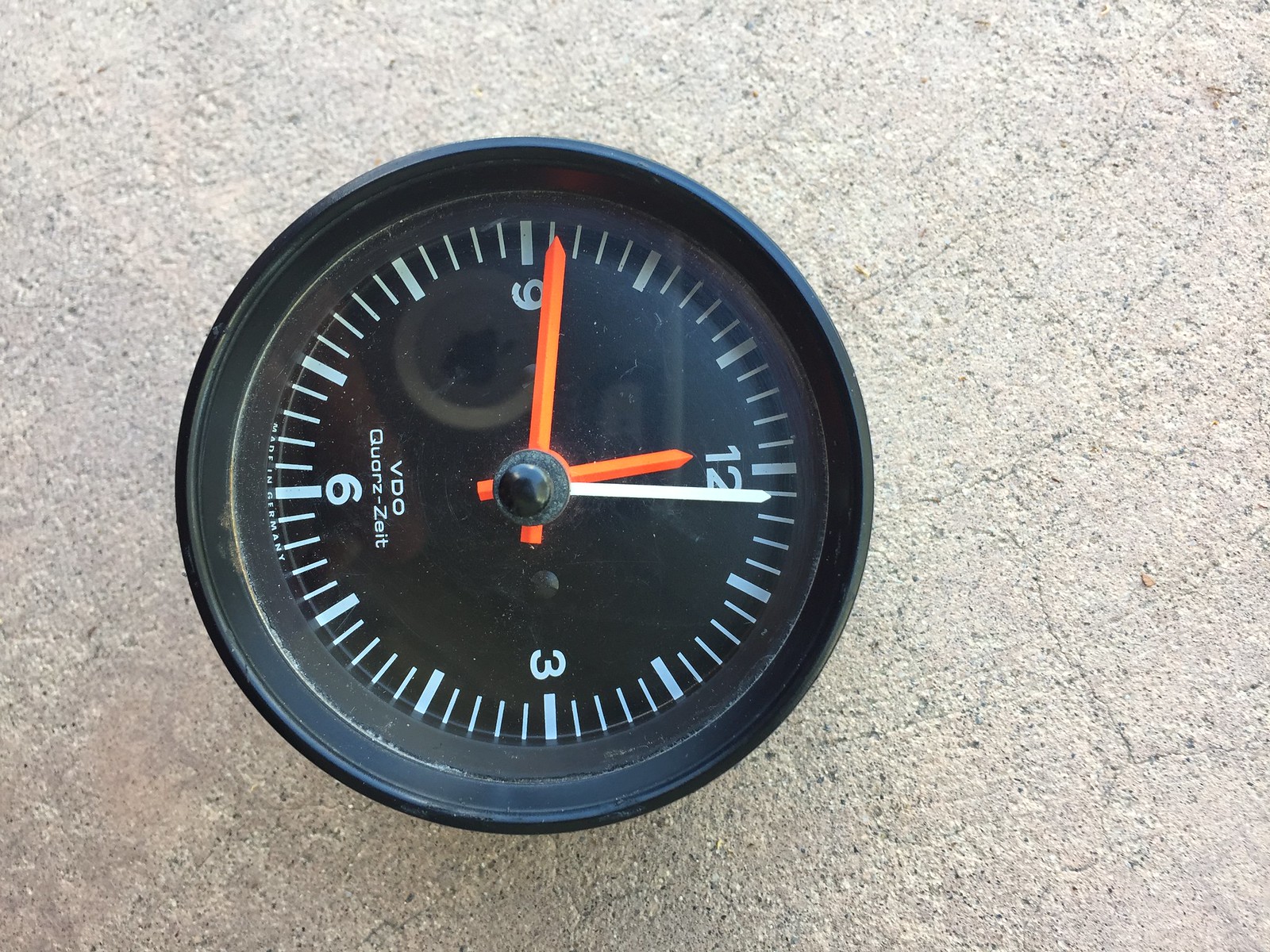This image captures a black gauge or clock face, centrally positioned yet turned slightly to the side, against a light gray concrete background with visible cracks and textures. The circular face features bold white numbers at the 12, 3, 6, and 9 positions, with smaller white dashes marking the intervals in between. Above the number 6, the text "VDO Quartz Zeit" is displayed in white. The clock has distinctive orange hour and minute hands, along with a white second hand, indicating a time of approximately 11:46. Three arrows point towards the numbers on the face, with two being orange and one white, adding to the intricate detail. Reflected on the clock's surface, an iPhone is visible, suggesting that someone is taking the photograph.